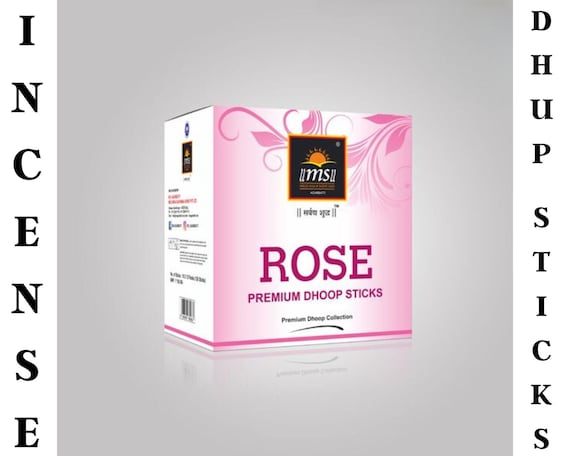This digital advertisement showcases a three-dimensional box set against a gray square background. The box itself features a pink front and white sides, creating a visually appealing contrast. The front of the box prominently displays the product name: "Rose Premium Dupe Stix." On the left side, the word "incense" is written in black text that runs vertically from top to bottom. Similarly, on the right side, the text "Dupe Stix, D-H-U-P, Stix" also appears vertically. At the bottom of the pink front panel, the phrase "Premium Dupe Collection" is elegantly inscribed, completing the sophisticated look of the package.